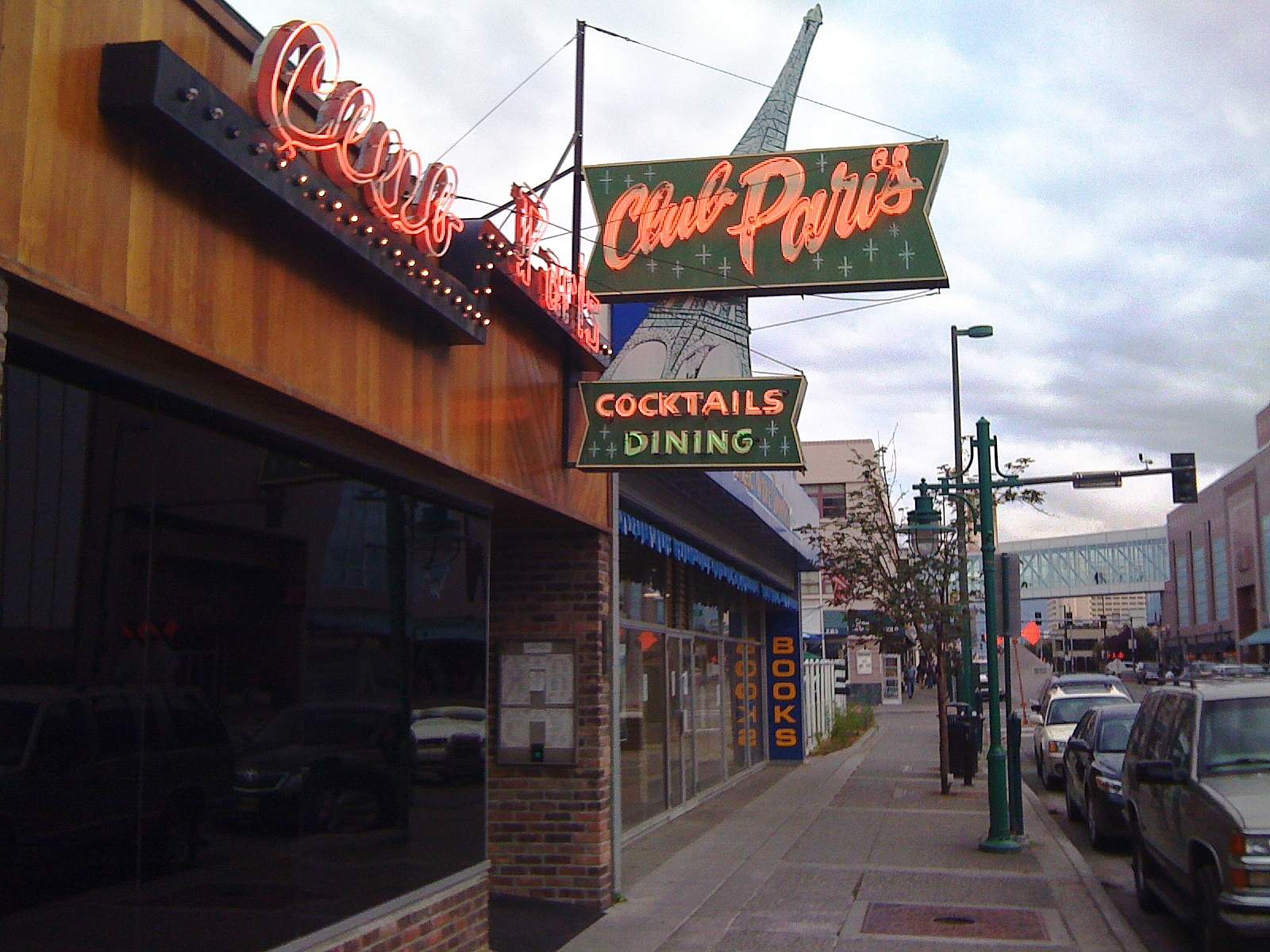The photograph depicts a bustling urban street scene during the daytime, framed horizontally at about six inches wide by four inches high. Dominating the left side of the image is a row of quaint small businesses, starting with a one-story building housing “Club Paris.” The sign for Club Paris is prominent, featuring orange text on a green background decorated with plus signs. Above the building, a smaller sign reads "Cocktails and Dining," with "Cocktails" in orange and "Dining" in green. The structure has a red brick façade, with a distinctive black-tinted front window shrouded in mystery, preventing a view of the interior.

To the right of Club Paris is a bookstore simply labeled "Books." The shops are situated next to a gray cement sidewalk edged with green streetlights. The street is flanked by parked cars, and an intriguing elevated bridge in the background connects two nearby buildings, hinting at a larger urban infrastructure. The sky is mostly covered in clouds, though bits of blue peek through on the left, adding a touch of color to the otherwise gray atmosphere.